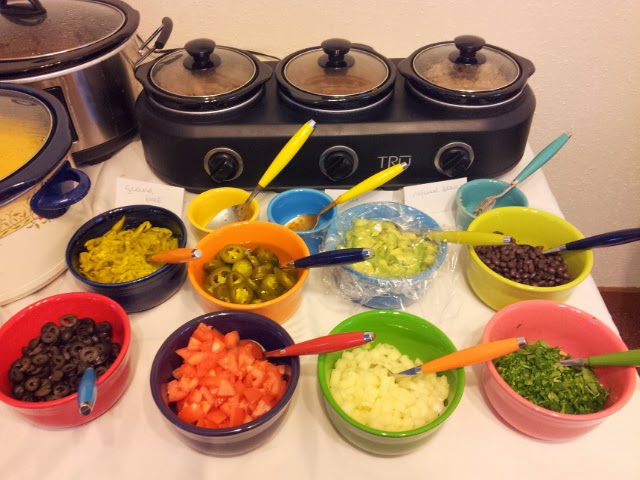This overhead photograph captures a lively nacho and taco party set on a white or off-white tablecloth, showcasing a variety of vibrant and mouth-watering elements. Dominating the back of the table is a silver-trimmed, buffet-style crock pot with three compartments labeled "True" in silver, flanked by knobs. In the upper left-hand corner, a large silver-colored crock pot with a steamed-up glass lid hints at the delicious contents inside. The left-center features a distinctive beige-colored crock pot adorned with a floral pattern and black trimmings, including the handles and lid edge. 

In the foreground, a colorful array of bowls is meticulously arranged, each containing a different topping for nachos or tacos. The toppings include sliced olives, diced tomatoes, diced onions, and freshly chopped cilantro. Sliced jalapeño peppers and pinto beans add to the variety, while a bowl of guacamole, thoughtfully covered with plastic wrap, promises extra flavor. The dark wooden floor peeks out from beneath the table, adding a touch of warmth to the scene, while a plain white wall in the background keeps the focus on the festive spread.